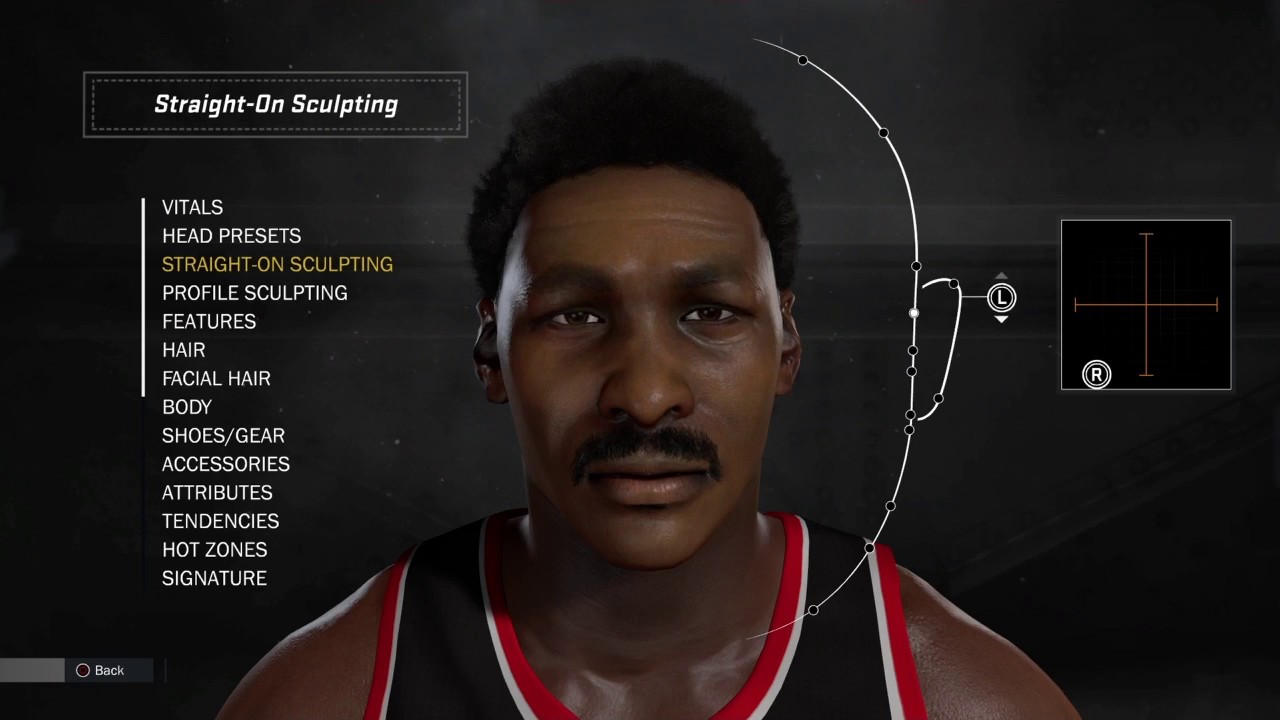The image showcases a highly realistic video game character creation screen, featuring a detailed portrayal of a Black male athlete with a medium afro and a mustache. He is wearing a black tank top with red accents. The character is depicted in a frontal view, gazing directly into the camera. To the right of the character's face, various cursor points and customization options for the ears are visible, indicating that users can hand-draw features to personalize their player's appearance. A crosshair and a box are also part of the interface.

The background is black, enhancing the focus on the character. The screen appears to be for an NBA-themed game, as suggested by the presence of a red 'B' button for PlayStation in the bottom left corner. The main customization option highlighted is "Straight On Sculpting," shown in white text with a dotted border and a solid border around it.

Below the main customization section, several other options are listed in white capitalized text: Vitals, Head Presets, Profile Sculpting, Features, Hair, Body, Shoes, Gear, Accessories, Attributes, Tendencies, Hot Zones, and Signatures. The current selection, "Straight On Sculpting," is highlighted in yellow. This comprehensive customization allows users to meticulously alter various aspects of their basketball player's appearance, including the eye shape, ear structure, and types of mustaches, such as cropped, tipped, thick, and pencil.